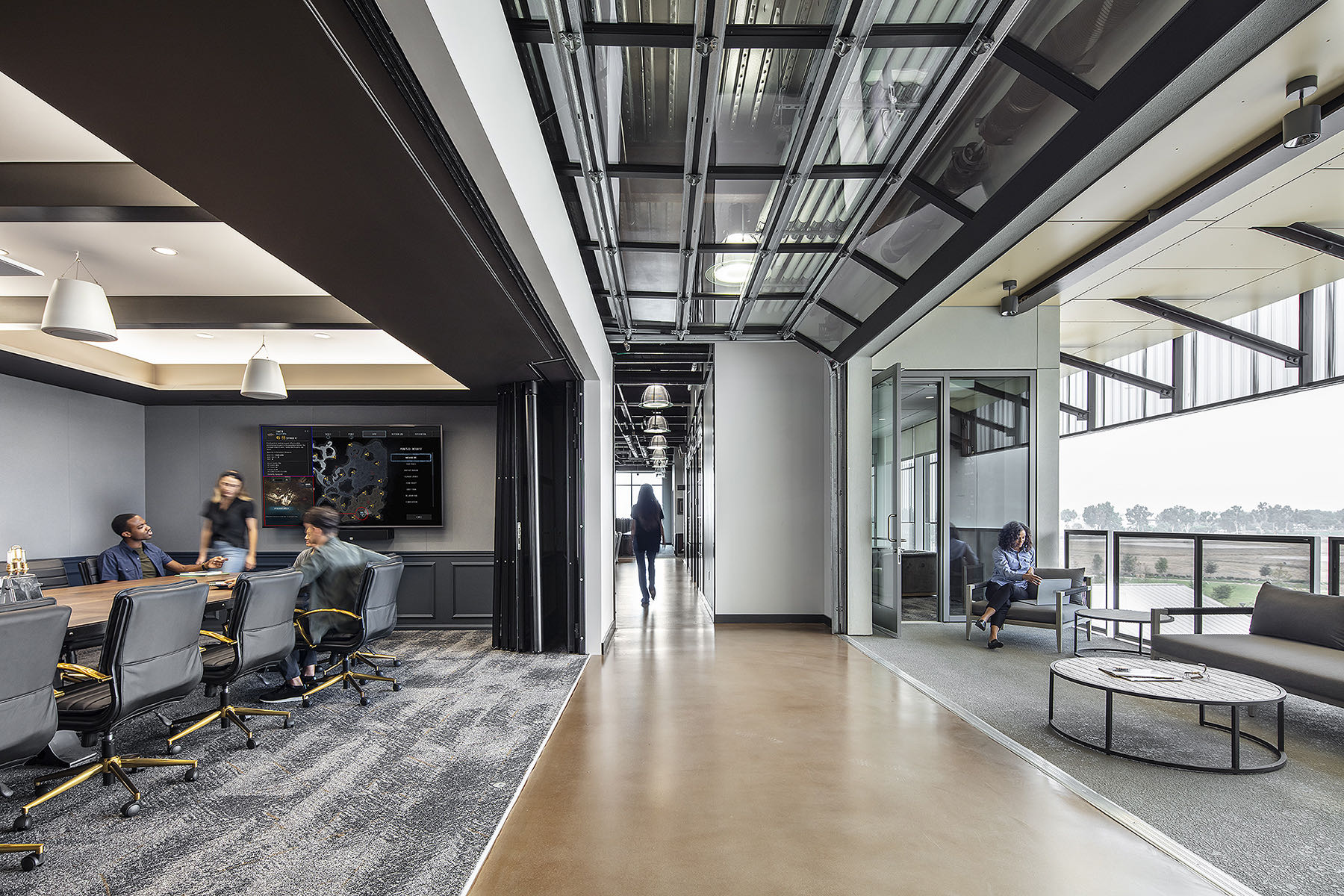The image depicts the interior of a modern office building characterized by its minimalist design and abundance of natural light. On the left-hand side of the image, there is a spacious conference room with a long brown table surrounded by black cushioned chairs accented with gold-colored metal. Seated at the table are two men, one on each side, while a woman stands at the head of the table, engaging with them. Behind her, mounted on the wall, is a television screen. The room features a gray and white rug beneath the table and is illuminated by white lights. 

To the right side of the image, a woman sits in a gray chair near a streamlined sofa, both of which are positioned by large windows that offer a view of an exterior balcony overlooking trees. She appears to be working on a laptop. The office design allows an open, airy feel, further enhanced by a glass and metal ceiling that spans the central corridor of the building. This corridor provides a clear line of sight through the office, and in the distance, a person is seen walking. Overall, the office space appears inviting and conducive to productivity, blending modern aesthetics with functional design elements.